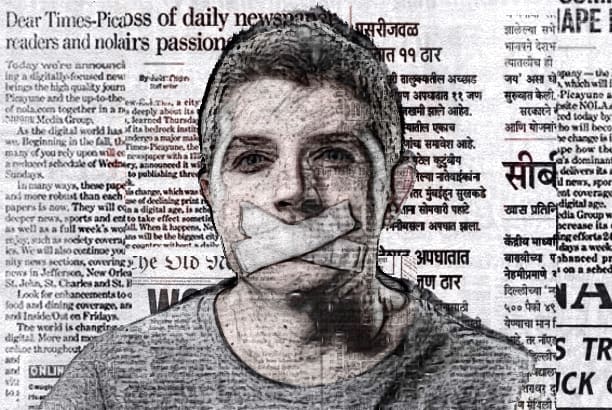The image is a black and white drawing of a young man, viewed from his shoulders to the top of his head. He has very short black hair, bushy eyebrows, and beady eyes, and he looks directly at the camera with a serious expression. The man is wearing a light-colored t-shirt, and his mouth is taped over with two pieces of tape forming an X. Behind him, there is a newspaper clipping, featuring text that includes phrases like "Dear Times" and "pick of daily news," written in English and another language. The newspaper serves as the backdrop for the image, suggesting a context of silencing or censorship, possibly related to a hostage situation. The overall composition conveys a sense of urgency and gravity.